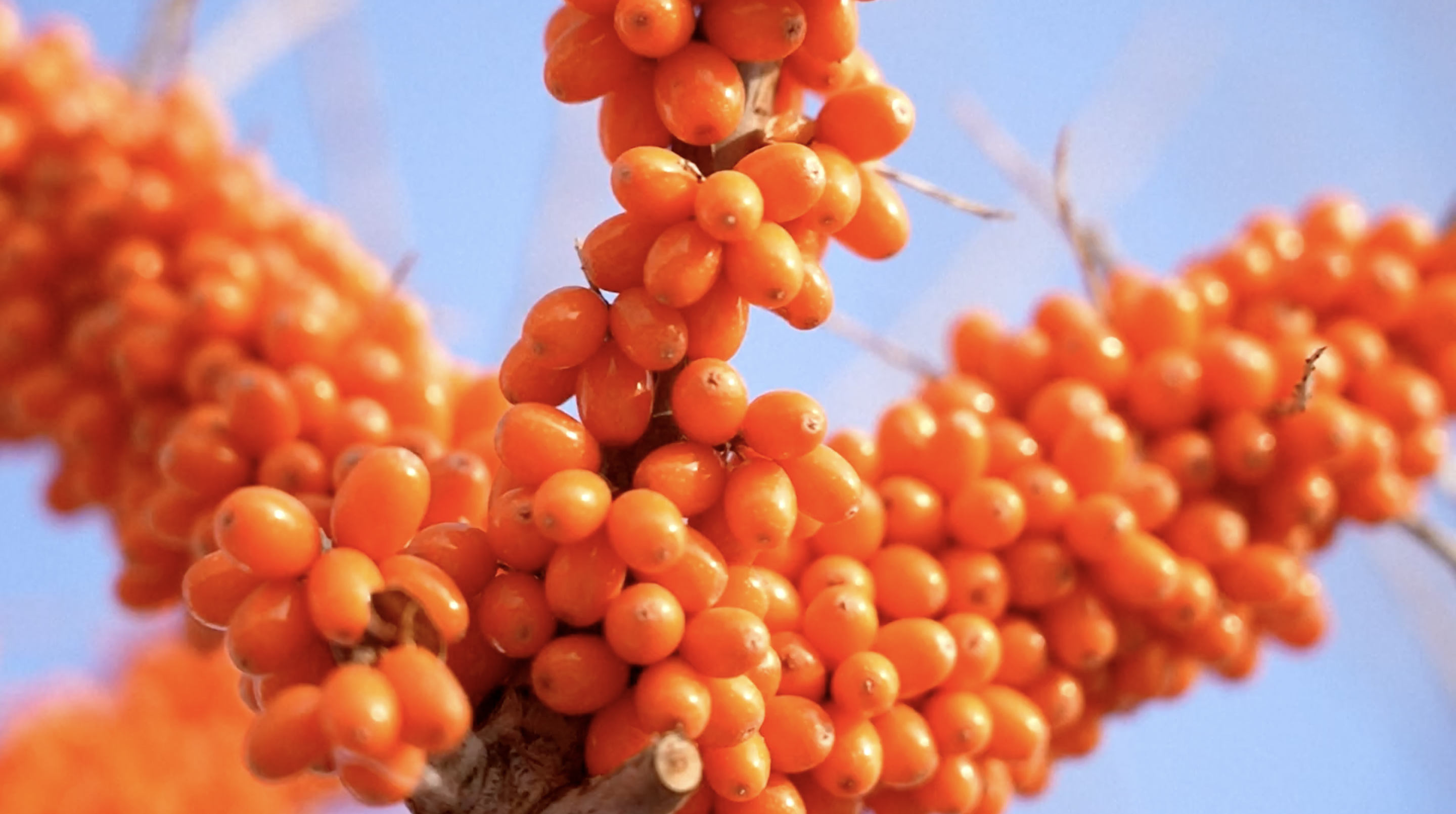This close-up image showcases a tree heavily laden with bright orange, oblong-shaped fruits or berries that resemble cherry tomatoes in size and shape. The berries densely cover three main branches, creating a near-total envelopment that only leaves a tiny bit of the wood of the branches visible, particularly in the bottom middle of the photograph. The image, a horizontal rectangle, is taken from an outdoor daytime setting, featuring a backdrop of a blurred, cloudless blue sky. The focus is sharp in the center where the thick branches, angling upward in different directions, and a thinner central branch meet, all adorned with scores of these vibrant berries. The numerous vivid orange fruits, some appearing almost reddish, contrast distinctly against the soft blue sky, capturing the eye's attention. The photograph's overall composition highlights the intricate clustering of fruits and the unique branching pattern, making for a visually striking and detailed scene.